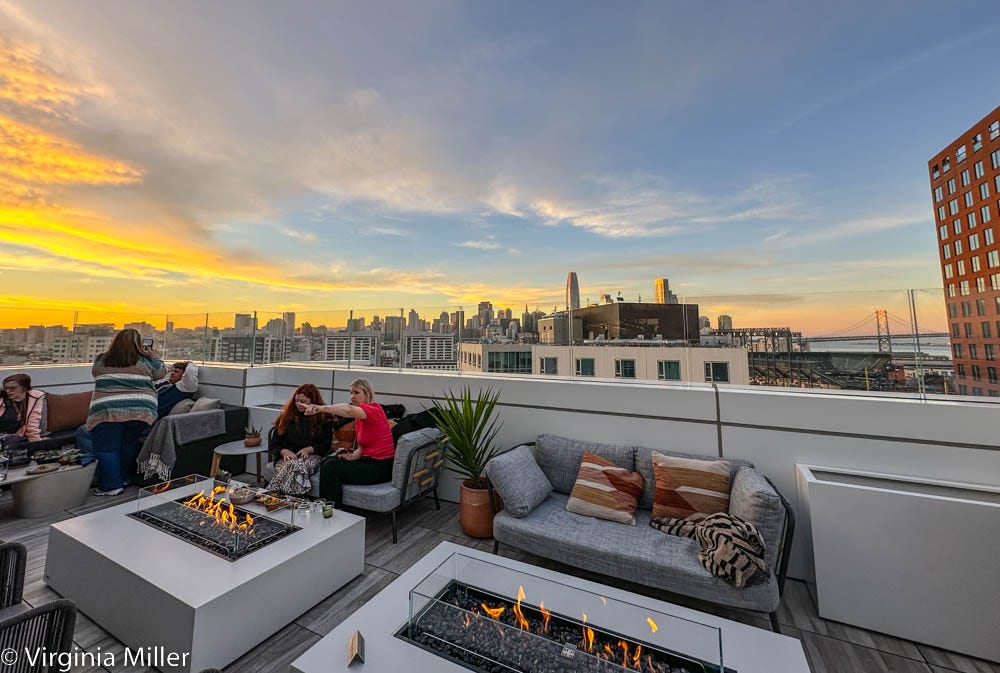This detailed color photograph, landscape-oriented, captures a vibrant rooftop lounge in a bustling city setting, emphasizing a harmony between urban atmosphere and a relaxing retreat. Spanning the bottom half of the image, the rooftop lounge is bordered by a light gray and white low wall. The flooring is a combination of gray wood decking and outdoor gray carpet. The centerpiece of the lounge is a comfortable seating area featuring gray couches adorned with a variety of throw pillows in blue, beige, and brick colors. 

In front of the couches are two raised, rectangular fire pits with gas flames flickering amidst gray rocks, each embedded in square white coffee tables, adding both warmth and visual appeal to the setting. People are casually seated on the couches, including a man in a red shirt pointing to something off-frame on the left, accompanied by a partially visible woman. To their left, a woman stands, gazing out over the cityscape of low-rise buildings that unfold beyond the lounge area.

The expansive sky above, transitioning from yellow and orange near the horizon to white and blue as it extends upwards, suggests either sunrise or sunset, casting a serene light over the scene. In the background on the right, a tall red brick building stands prominently among shorter structures. In the bottom left corner, a copyright mark reads "© Virginia Miller." The photograph, with its realistic depiction, evokes a sense of warmth and relaxation amid urban surroundings.